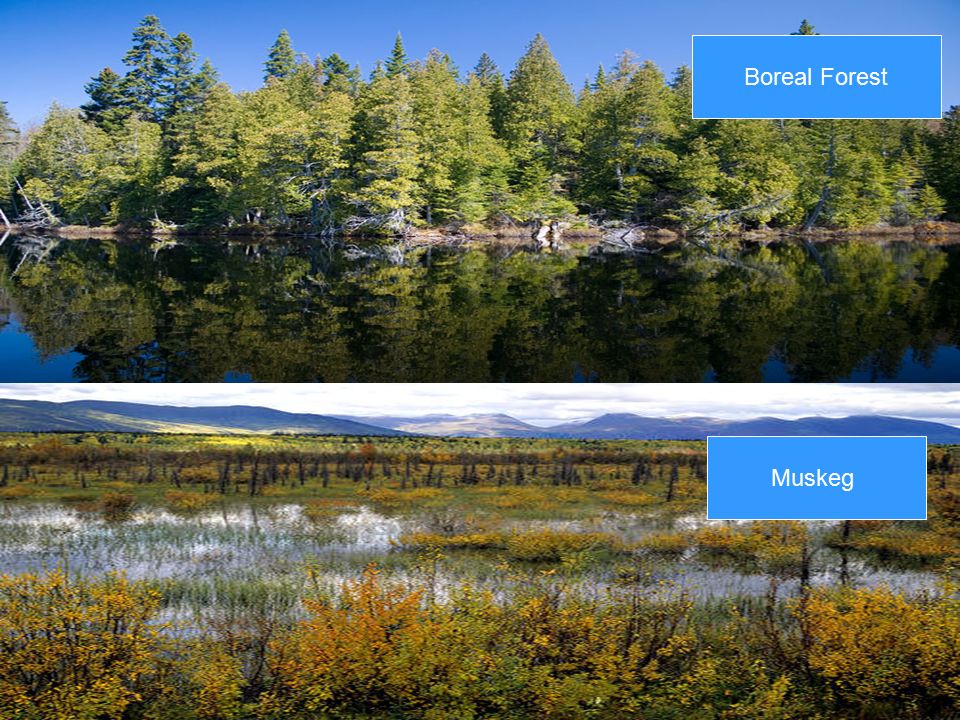The image is split into two long rectangular sections, each depicting a different forest ecosystem with a distinct blue label in white text. The top image, labeled "Boreal Forest," is a serene daytime scene featuring a calm lake that perfectly mirrors a line of stately, old pine trees in the background. The sky is a vivid, bright blue, enhancing the tranquility of the reflective water. The bottom image is labeled "Muskeg" and presents a more swampy or marshy landscape. Here, flat green areas are interspersed with patches of water and wild bushes displaying little orange and yellow leaves. In the distance, a line of mountains looms under a sky filled with clouds seemingly touching the peaks. The overall color palette is richly natural, highlighting the greens of the foliage, the blues of the sky, the grays of the mountains, and the whites of the clouds, making both images strikingly beautiful and evocative of their respective environments.